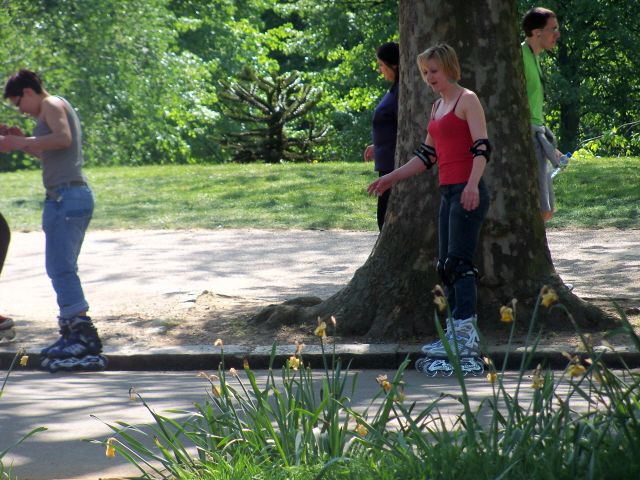In this vibrant park setting teeming with greenery, the foreground features a cluster of yellow daffodils, adding a splash of color to the scene. Dominating the middle of the image is a large tree with a prominently visible trunk surrounded by dirt. Behind this tree, the background reveals a lush expanse of grass dotted with several trees and bushes.

The image captures four people amidst this serene environment. In front of the tree, a man and a woman are engaged in rollerblading along a pathway. The man, dressed in a gray tank top and blue jeans, glides effortlessly without any protective gear. Beside him, the woman, in a red tank top and black jeans, is equipped with elbow and knee pads but notably lacks a helmet. Her gray rollerblade boots are evident, suggesting she is just starting off on her rollerblades. 

Behind the tree, partially obscured, stand two more individuals. One is a woman wearing a blue shirt and dark-colored pants, and the other is a man clad in a green shirt with gray shorts, with something possibly tied around his waist. Their positions make it unclear whether they are also on rollerblades, but they add to the overall activity and interaction within this picturesque park scene.